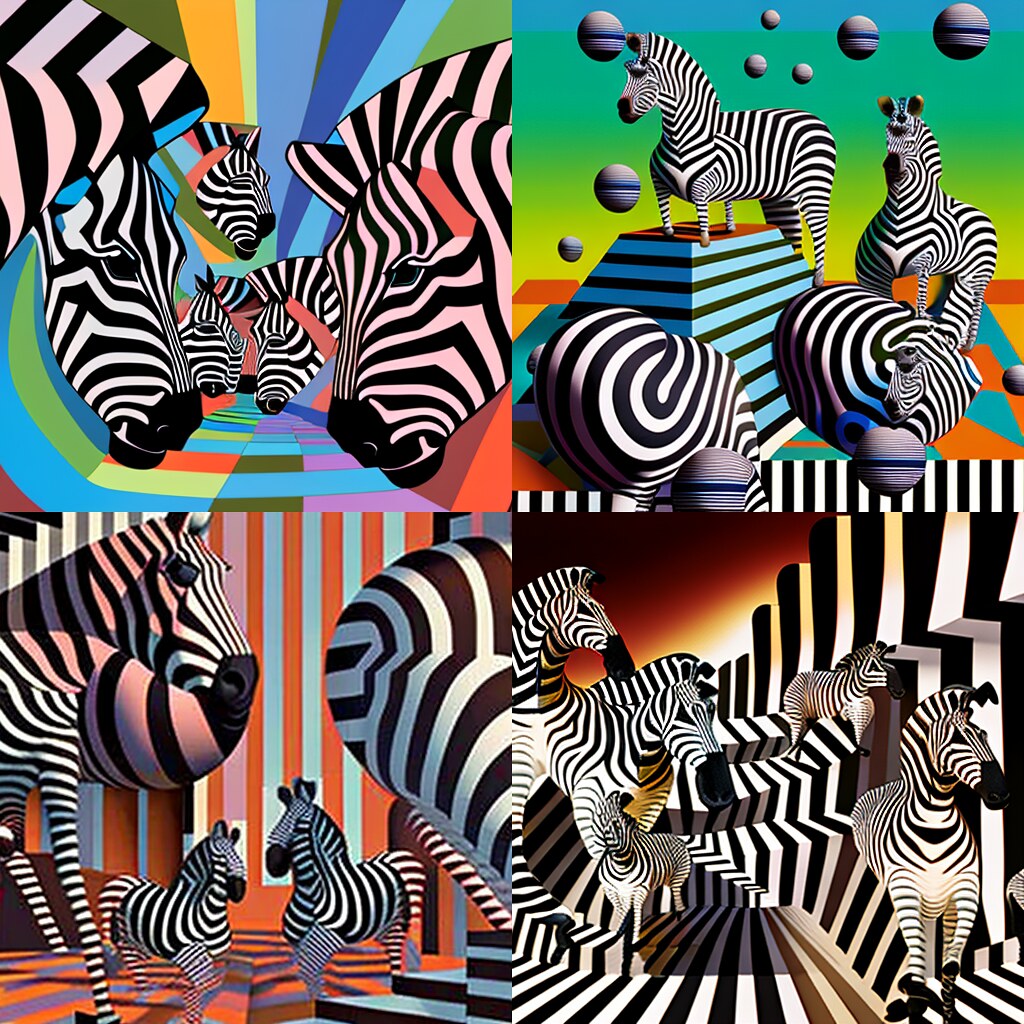This modern and abstract image features a square composite of four smaller square panels, arranged in a 2x2 grid, each illustrating surreal, computer-animated scenes with zebras. The artistic, edgy style and vibrant colors create a geometric and modern art vibe, reminiscent of the work of M.C. Escher with its surreal, 3D effects and intricate patterns. 

The top left panel showcases a dynamic array of five zebras amidst a flurry of yellow, green, and blue stripes. The top right panel is a vibrant display with a scenic horizon, filled with various colorful shapes, white balls, and a blue-and-black triangle on which two zebras stand pyramid-style. In the bottom left panel, three zebras—alongside zebra-like patterns—appear amid vertical orange and light blue stripes, creating a bewildering effect of what is zebra and what is not. The bottom right panel features a striking contrast of black and white zebras standing on similarly colored platforms against a striking red sky. Each panel uniquely utilizes the zebra pattern, adding to the surreal and mesmerizing quality of the image.